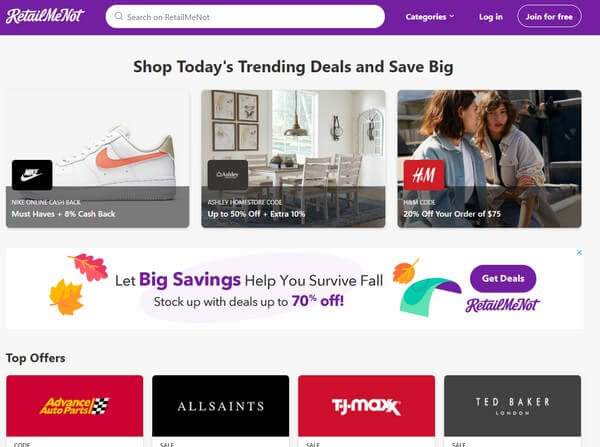This image showcases an online shopping website with a focus on deals and promotions. The top of the webpage features a prominent purple navigation bar with the logo "RetailMeNot" on the left, accompanied by a white search bar to the right. Options for "Categories," "Login," and "Join for Free" are also present on this bar.

Beneath the navigation bar, the page has a clean white background with a header in bold black text that reads, "Shop Today's Trending Deals and Save Big." Below this header, there are three distinct images representing trending deals:

1. A high-quality image of a white Nike sneaker with an orange swoosh, pointing to the left. The Nike logo is noticeable in black at the lower left of this section.
2. A stylish interior shot of a dining room with the label "Ashley Furniture" showcasing their offerings.
3. A picture of two women engaged in conversation with the label "H&M," indicating deals available at this store.

Further down, there is a large white banner adorned with a fall leaf design, promoting significant seasonal savings. The text on the banner reads, "Let Big Savings Help You Survive Fall. Stock Up with Deals Up to 70% Off." A purple oval button on the right side of the banner invites users to "Get Deals," and below this button, the "RetailMeNot" brand is mentioned again.

At the bottom of the image, there are four horizontal rectangles highlighting top offers from various retailers:
- The first rectangle, depicting "Advance Auto Parts," is designed with a focus on automotive deals.
- The second rectangle, in black with white text, features the fashion retailer "AllSaints."
- The third rectangle is bold red with "TJ Maxx" written in white, emphasizing discounted fashion and home goods.
- The last rectangle, with a grey background, showcases "Ted Baker London," indicating high-end fashion deals.

Overall, this webpage is visually organized and designed to attract customers to the latest deals and promotions available on "RetailMeNot."